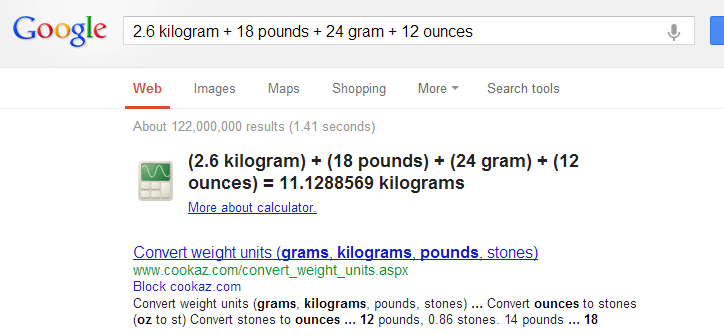The image is a screenshot of a Google search results page. At the top, there is a gray navigation bar with the Google logo on the left side. The logo displays the word "Google" in its distinctive multi-colored scheme: the capital 'G' and lowercase 'g' in blue, the first 'o' and 'e' in red, the second 'o' in yellow, and the 'l' in green. Next to the logo is a white search bar with a small microphone icon on its right side, indicative of the voice search feature. Adjacent to the search bar, partially visible, is what appears to be a blue button.

Within the search bar, the user has entered the query: "2.6 kilogram plus 18 pounds plus 24 gram plus 12 ounces." Below the search bar is a secondary navigation bar with selectable tabs labeled "Web," "Images," "Maps," "Shopping," and a dropdown menu option "More," alongside "Search tools." The "Web" tab is currently selected.

The results page indicates approximately 122 million results found in 1.41 seconds. Prominently displayed under this information is a calculator icon with the calculation: "2.6 kilogram plus 18 pounds plus 24 gram plus 12 ounces equals 11.1288569 kilograms." Below this calculation, a line of text reads: "convert weight units, grams, kilograms, pounds, stones," with a web address included: www.cookas.com/convert_weight_units.aspx.